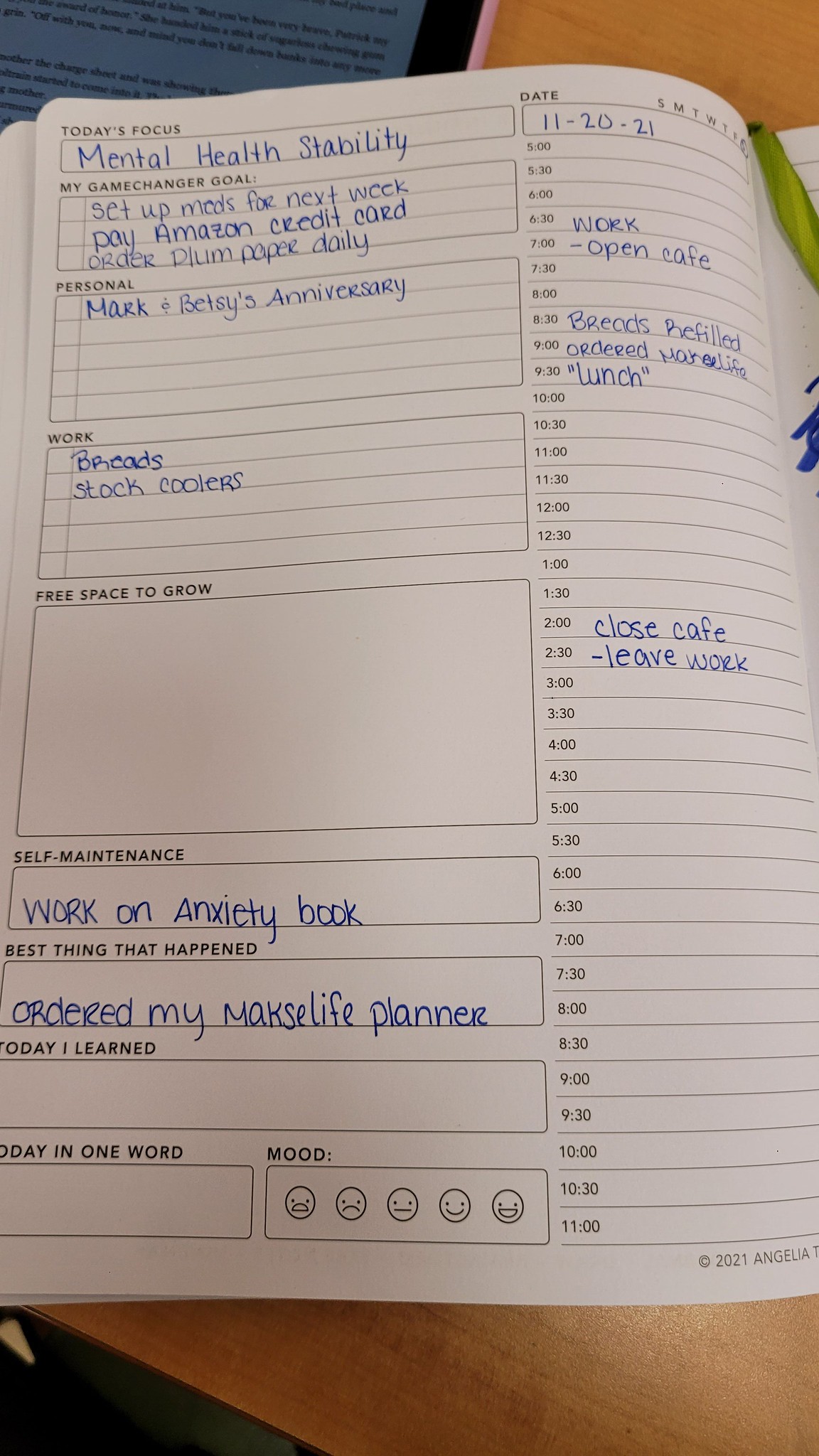This color photograph captures a neatly arranged scene on a wooden desk, where the wood grain subtly lends texture to the background. Positioned centrally is an open notebook, prominently featuring a page with detailed plans. At the top of the notebook page, underlined in blue ink, is the heading "Today's Focus," emphasizing "Mental Health Stability." Below, the page is segmented into various sections, each meticulously filled out. 

The "My Game Changer Goal" section lists tasks such as "Set up meds for next week," "Pay Amazon Credit Card," and "Order Plum Paper Daily." The "Personal" heading notes "Mark and Betsy's Anniversary," while the "Work" section mentions tasks like "Breads" and "Stock Coolers." In the "Self-Maintenance" box, an entry reads, "Work on Anxiety Book." 

Additionally, the "Best Thing That Happened" section highlights, "Ordered my Makes Life Planner." To the right of these entries, a detailed daily schedule is organized in half-hour increments, starting with "Work" at 6:30, followed by "Open Cafe" at 7:00, "Breads Refilled" at 8:30, "Ordered Max Life" at 9:00, "Lunch" at 9:30, "Closed Cafe" at 2:00, and "Leave Work" at 2:30. Furthermore, in the top left corner of the desk lies another piece of paper, though its text remains indistinct.